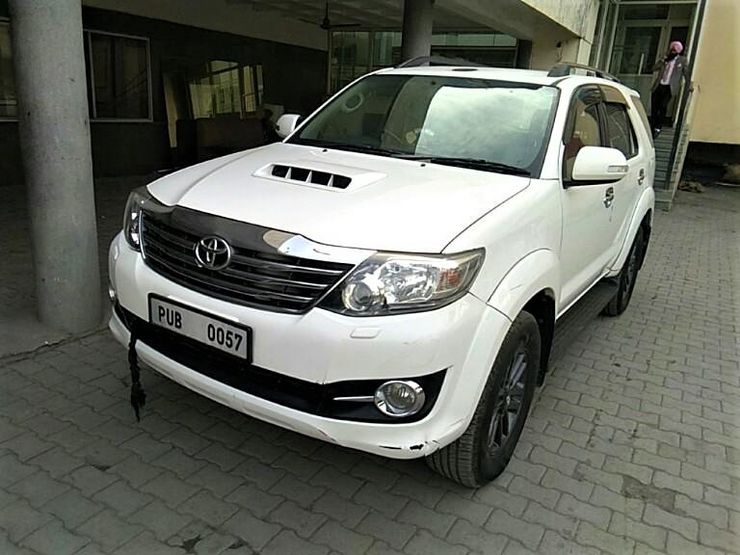In the photograph, a large white SUV-style car, strikingly positioned in the center, dominates the scene. The SUV is parked on a stone or paved concrete surface, oriented at a slight diagonal angle that allows both the front and side views of the vehicle to be visible. It stretches across much of the image, occupying roughly 70% of the frame from the bottom to the top.

The surroundings include a few concrete pillars and a building with glass windows that cast subtle reflections in the background. Although slightly obscured by dim lighting, the building suggests an office-like environment with its neutral colors and structured design. Additionally, to the right of the SUV stands a set of steps leading up to a door, which is a dark green color, contrasting with the cream-colored exterior of the building.

A person, small in the context of the photo but noticeable, stands on these steps. The individual appears smartly dressed, possibly in a suit, with features that hint at a pink turban and gray blazer, indicating a formal attire. 

There's no additional text in the image except for the car’s personalized number plate, marked with "PUB 0057." The photograph appears to be taken outdoors, capturing a quiet, structured scene bathed in natural daylight, potentially during mid-day.